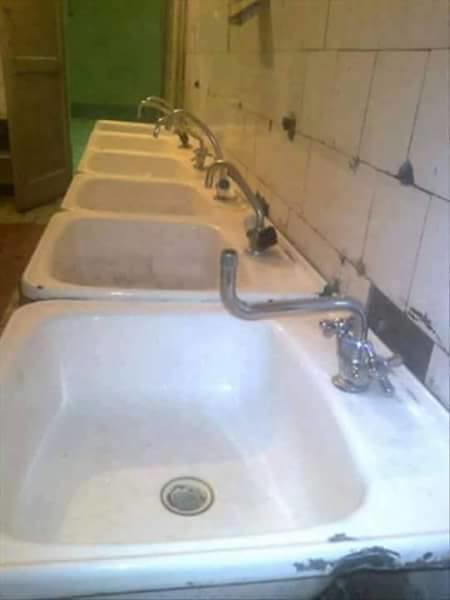The image captures an aged public restroom, likely within an institutional facility such as a school, penitentiary, or detention center. The focal point is a row of six cast enamel single-basin sinks, aligned under an old, cracked, and dirty white tile wall. The tiles, approximately eight inches square, are staggered, with numerous missing pieces and large, gaping holes where a mirror once was. The wall and tiles are marred with black spots and signs of mold, contributing to the overall sense of neglect.

The foreground sink, prominently larger due to the camera angle, shows significant wear with extensive chipping, exposing the underlying metal and even having a chunk missing. The simple arced faucets are equipped with old-style cross handles for hot and cold water, though the faucet of the nearest sink has been tampered with, bent upwards in a prankish manner, suggesting that activating it would spray water upwards rather than into the basin.

As the line of sinks recedes in perspective, they diminish in size, converging towards an open brown door at the back of the photo. Beyond the door lies a greenish hallway with a narrow walkway, adding an additional layer of institutional ambience to the scene. The overall rugged and utilitarian appearance of the area evokes a sense of heavy usage and poor maintenance, characteristic of facilities that must accommodate large volumes of people daily.